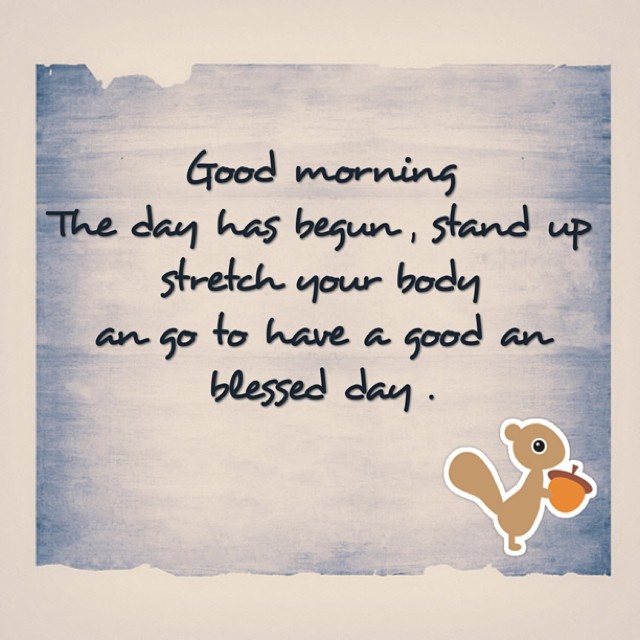This image is an inspirational graphic designed to look like a poster. It features a light gray border forming a frame around a textured blue background, which is lighter in the center, almost white, and darkens towards the edges. The blue edges appear to have chunks missing, giving a worn effect. In the bottom right corner, there is a sticker of a cartoon squirrel with a black eye, holding a gold and brown acorn, outlined in white as if it's a child's sticker. The poster displays five lines of black cursive text, styled to appear handwritten but actually printed, saying: "Good morning. The day has begun, stand up, stretch your body, and go have a good and blessed day." Notably, the word "and" is misspelled, with a missing 'd'.